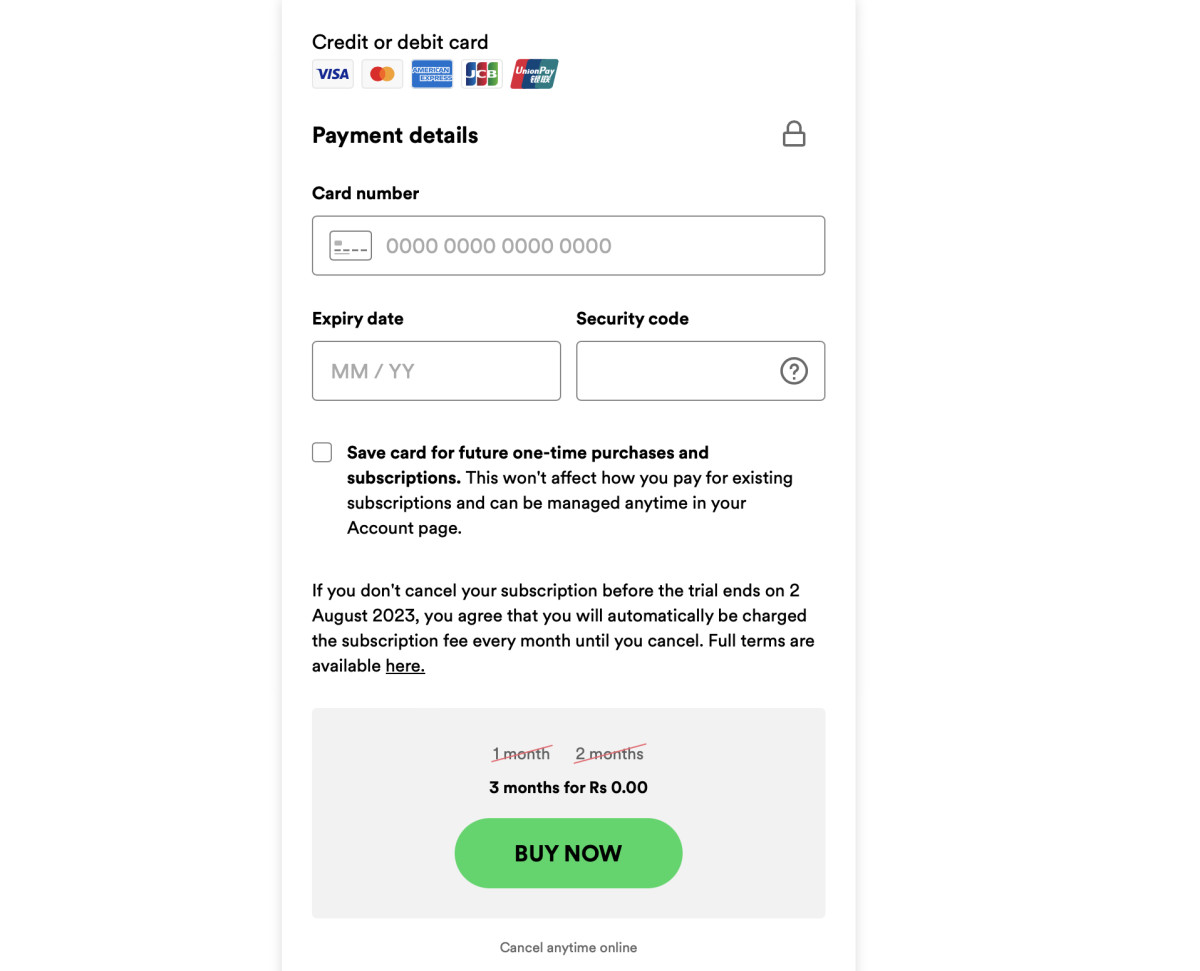This is a detailed screenshot depicting the payment page of an app, likely viewed on a smartphone. The background is predominantly white for a clean interface. 

At the top, bold text reads "Credit or Debit Card," flanked by symbols for Visa, MasterCard, American Express, and two additional payment methods, indicating accepted card types. Below, prominent text stating "Payment Details" is aligned to the left, accompanied by a secure lock icon on the right, emphasizing security.

The section that follows contains various forms for card information. First, there is a labeled box for the card number. Directly below, there are fields for the card's expiry date, split into month and year. Positioned to the right of this is a box for the security code, accompanied by a circle containing a question mark to offer help or additional information.

Under these fields, a checkbox option titled, "Save card for future one-time purchases and subscriptions," offers users the convenience of saving their card details. It is followed by a clarifying note that reads, "This won't affect how you pay for existing subscriptions and can be managed anytime in your account page."

Further below, a warning message informs users, "If you don't cancel your subscription before the trial ends on 2 August 2023, you agree that you will automatically be charged the subscription fee every month until you cancel." This message is accompanied by a hyperlink labeled "Full terms are available here" for users who wish to read the full terms and conditions.

At the bottom of the screenshot, a light gray rectangular box displays subscription offers, with "One month" and "Two months" options crossed out in red. Next to these, a special offer reads, "Three months for ₹0.00," enticing users with an extended trial period. Adjacent to this offer is a prominent green button labeled "Buy Now." Below this button, the text "Cancel anytime online" reassures users of their right to cancel the subscription without hassle.